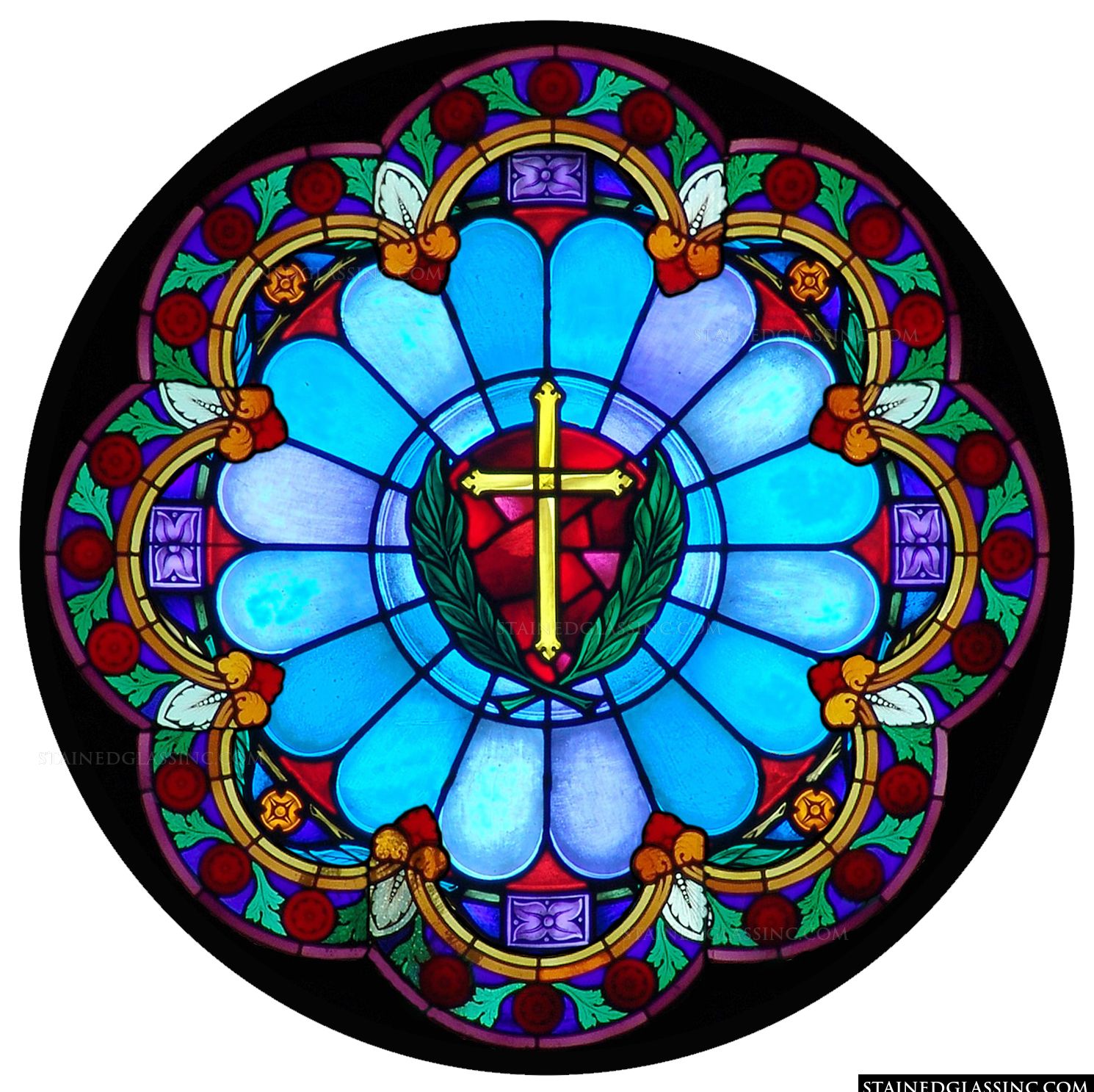This image presents a circular stained glass window, abundant with intricate details and vivid colors, evocative of traditional Catholic church designs. At the center, a prominent gold cross is encircled by two olive or laurel leaves, symbolizing peace and victory. The backdrop behind the cross is a rich red, providing a striking contrast. Radiating outward, the design mimics a flower, reminiscent of a zinnia, with petal-like segments transitioning from sky blue to light violet hues. These petals are interspersed with red sections, enhancing the floral motif.

The outer part of the stained glass showcases ornate floral elements featuring vibrant oranges and abstract shapes that resemble shields. Additional decorative motifs include leaves and small abstract red circles, possibly representing roses, seamlessly blending with the petal design. The window’s edge is adorned with more intricate patterns in shades of white, yellow, blue, and green, completing the elaborate floral arrangement.

At the bottom of the image, a website name, "StainedGlassing.com," is visible in white font against a black background, suggesting either the creator's portfolio or a representation of their work. The harmonious interplay of colors—blues, reds, violets, purples, and gold—enhances the window's beauty, making it a vibrant and visually captivating religious piece.